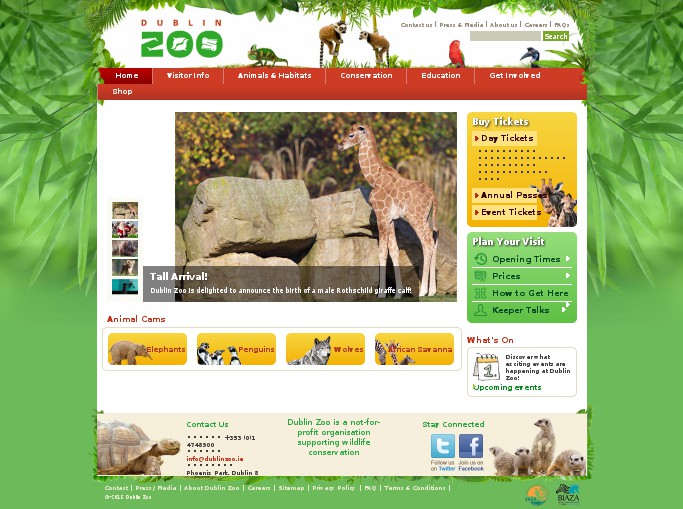The screenshot of the Dublin Zoo website features a light green border decorated with subtle, long and narrow tree leaf drawings on the top left and right corners. At the center, there's a white square area comprising the main content. The header graphic, with a white background, showcases "Dublin Zoo" on the upper left — the word "Zoo" is in green font. To the right of the header, small illustrations of animals including a couple of monkeys, a red parrot, and a green lizard add a touch of whimsy. Underneath the header, there's a brick red menu bar with white font displaying various navigation options from left to right: "Home," "Visitor Info," "Animals and Habitats," "Conservation," "Education," and partially visible "Getting...". Dominating the central part of the page is a large photograph featuring a baby giraffe standing on the left side next to four large boulders.